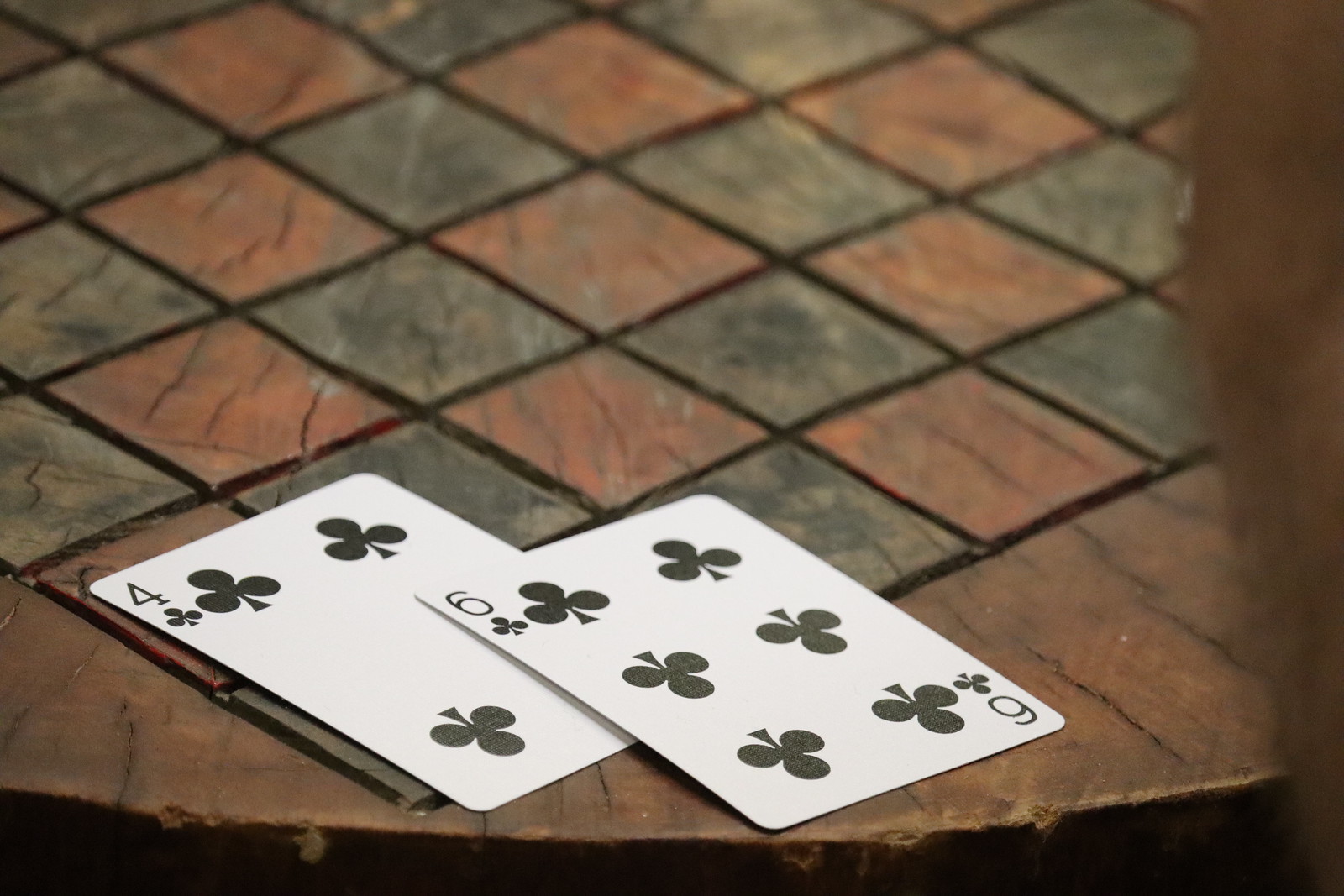In this photograph, two pristine playing cards—the Four of Clubs and the Six of Clubs—are casually placed, with the latter overlapping the former. The cards, not marred by stains or frayed edges, lie on an old, round gaming table. The table features a carved and painted red-and-green checkerboard or chessboard design, though its age is evident from the chips around the edges, numerous scratches, and faded paint. The scene captures a contrast between the well-kept cards and the worn table. On the far right of the image, a blurred sliver of an arm intrudes slightly, adding a hint of human presence without diverting attention from the central elements. The cards show minor buckling, likely from use, but remain in overall good condition.